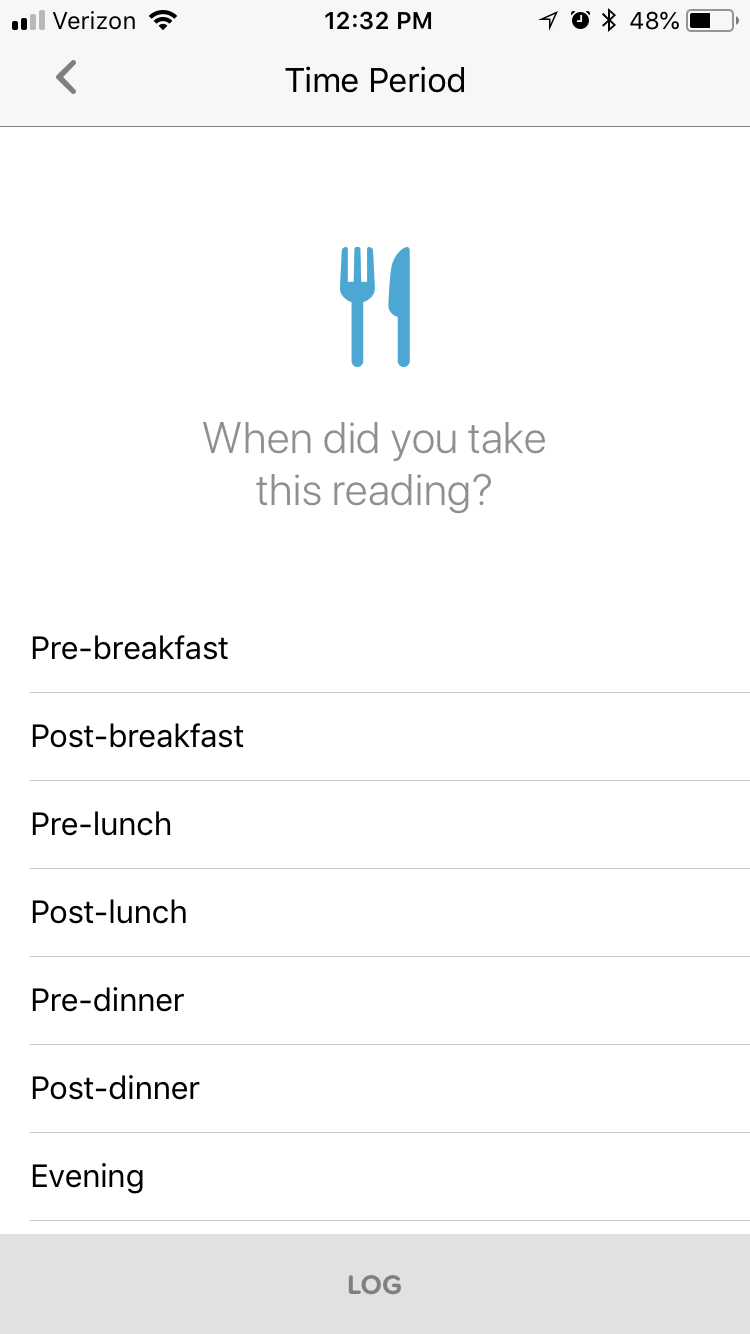The image displayed on the smartphone screen is from a blood glucose monitoring app. Across the top, there is a thick pale gray bar featuring black text. On the top left, there is a signal bar icon followed by the carrier name "Verizon" and the Wi-Fi icon. Centered at the top is the current time displayed as "12:32 p.m." On the right, there is a row of icons indicating Bluetooth connectivity and battery charge status.

Beneath the time, the rest of the screen predominantly displays a white background. At the top of this section, there is a bright blue illustration of a fork and knife. The fork has three tines, and both utensils are rendered in a solid blue color without any outlines.

Below the illustration, the text reads, "When did you take this reading?" in gray letters. This phrase is followed by a list or chart detailing different meal-related time periods for blood glucose readings, written in bold, black Arial typeface. The specific times include pre-breakfast, post-breakfast, pre-lunch, post-lunch, pre-dinner, post-dinner, and evening, each underlined with a thin gray line.

At the bottom, there's a long gray button labeled "Log," indicating where users can enter and save their glucose readings. While it is not explicitly mentioned, it seems evident that this interface is used for tracking blood sugar levels pre- and post-meal.